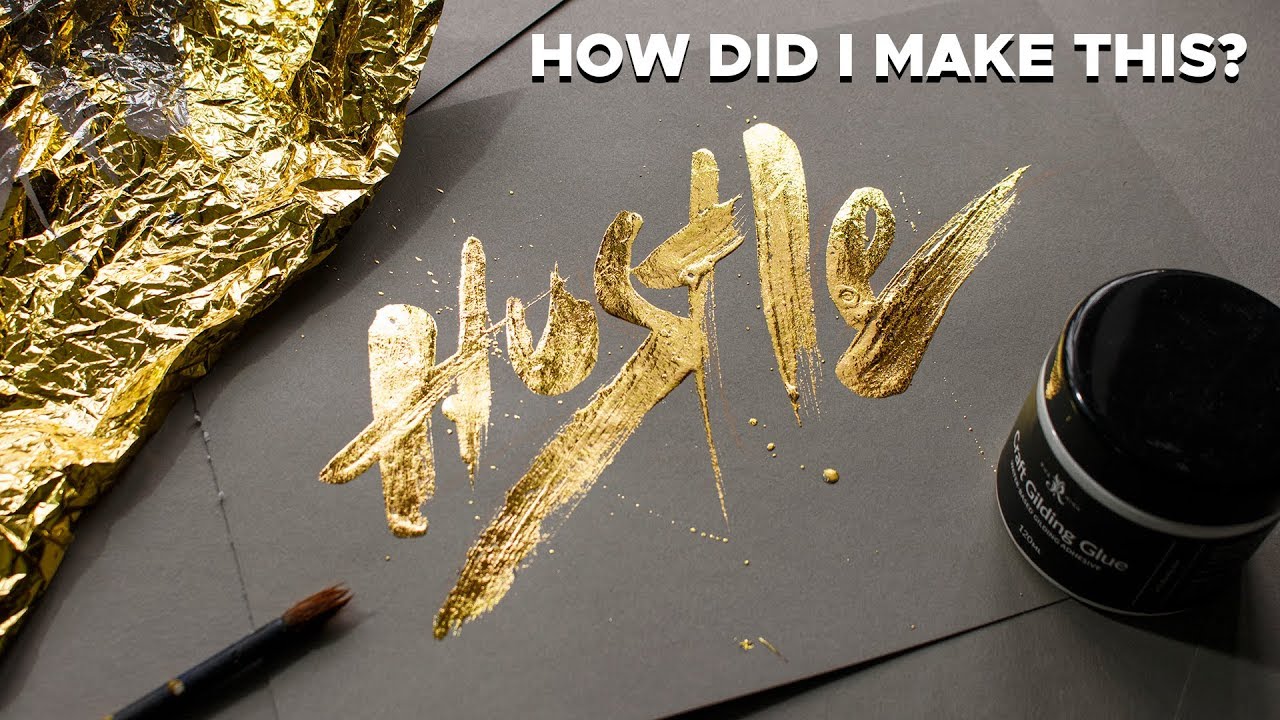This image displays a creatively designed postcard-sized piece of art with a distinct, hand-crafted feel. The background of the card features a flat, light gray construction paper material. Prominently in the center, the word "HUSTLE" is written in a stylish, finger-painted font using gold foil or gold metallic paint, showcasing slight dribbles and drips from the 'L' and 'T'. The texture of the paint gives a dynamic and textured appearance, with splatters of gold paint adding to the artistic realness. The top right-hand corner of the card bears a bold, white text outlined in black that reads, "HOW DID I MAKE THIS?" This text is right-aligned and heavily shadowed for emphasis. In the upper left corner, a crinkled piece of gold foil extends diagonally across part of the card, its wrinkles casting shadows and adding depth. In the lower portion of the image, a black-handled paintbrush sits on the left, while a black inkwell or glue pot is positioned on the right, suggesting the tools used in creating this intricate piece.